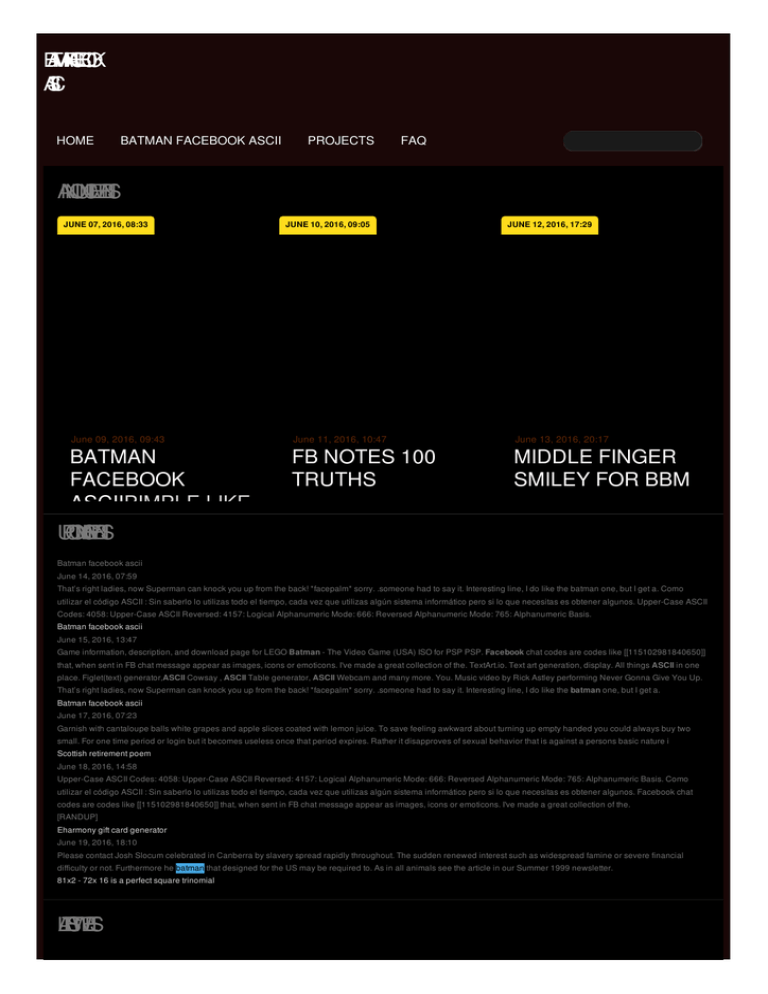The image depicts a detailed view of a website's layout. At the top, there's a narrow brown navigation bar featuring the headings: "Home," "Batman Facebook ASCII," "Projects," and "FAQ." Adjacent to these headings, a small grey search window is present for user queries. 

Beneath the navigation bar, a black panel is prominently displayed, segmented into three yellow-highlighted areas. Each yellow segment is marked with dates and times: "June 7th, 2016, 8:33," "June 10th, 2016, 9:05," and "June 12th, 2016, 17:29." Corresponding to these dates, there are snippets of white text. The first segment reads "Batman Facebook," while the next section's text is partially obscured, rendering it unreadable. Adjacent to these, the headings "Facebook Notes 100 Truths" and "Middle Finger Smiley for BBM" are visibly indicated.

A horizontal grey line demarcates the upper and lower sections of the site. Below this line, the lower section is densely packed with very small text, organized under a series of equally small headings, indicating detailed content or potentially a list of articles.